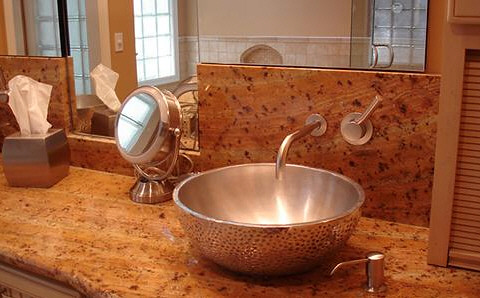This image features a meticulously designed modern bathroom. Dominating the foreground is a large mirror that spans the width of the bathroom, reflecting the sophisticated details of the interior. Below the mirror sits a sleek countertop accompanied by a distinctive backsplash that resembles a blend of light and dark brown cork, interspersed with delicate flecks of white. A stylish tissue holder, merging elements of silver and bronze, holds a crisp white tissue.

Adding to the elegance of the bathroom is a prominent double mirror mounted on a silver stand, which commands attention with its exquisite and substantial design. The centerpiece of the countertop is a unique silver sink resembling a large, knotted bowl; its exterior has a textured finish, while the interior boasts a smooth metal surface. This is complemented by a silver tap and a built-in soap dispenser, all contributing to the cohesive metallic theme.

A small brown louvered door adds a touch of warmth and rustic charm to the setting. Reflected in the expansive mirror, one can see the entrance to a spacious walk-in shower, adorned with a sizeable white window alongside another window that allows ample natural light to flood the room. Overall, this bathroom epitomizes a blend of modern aesthetics and functional elegance.